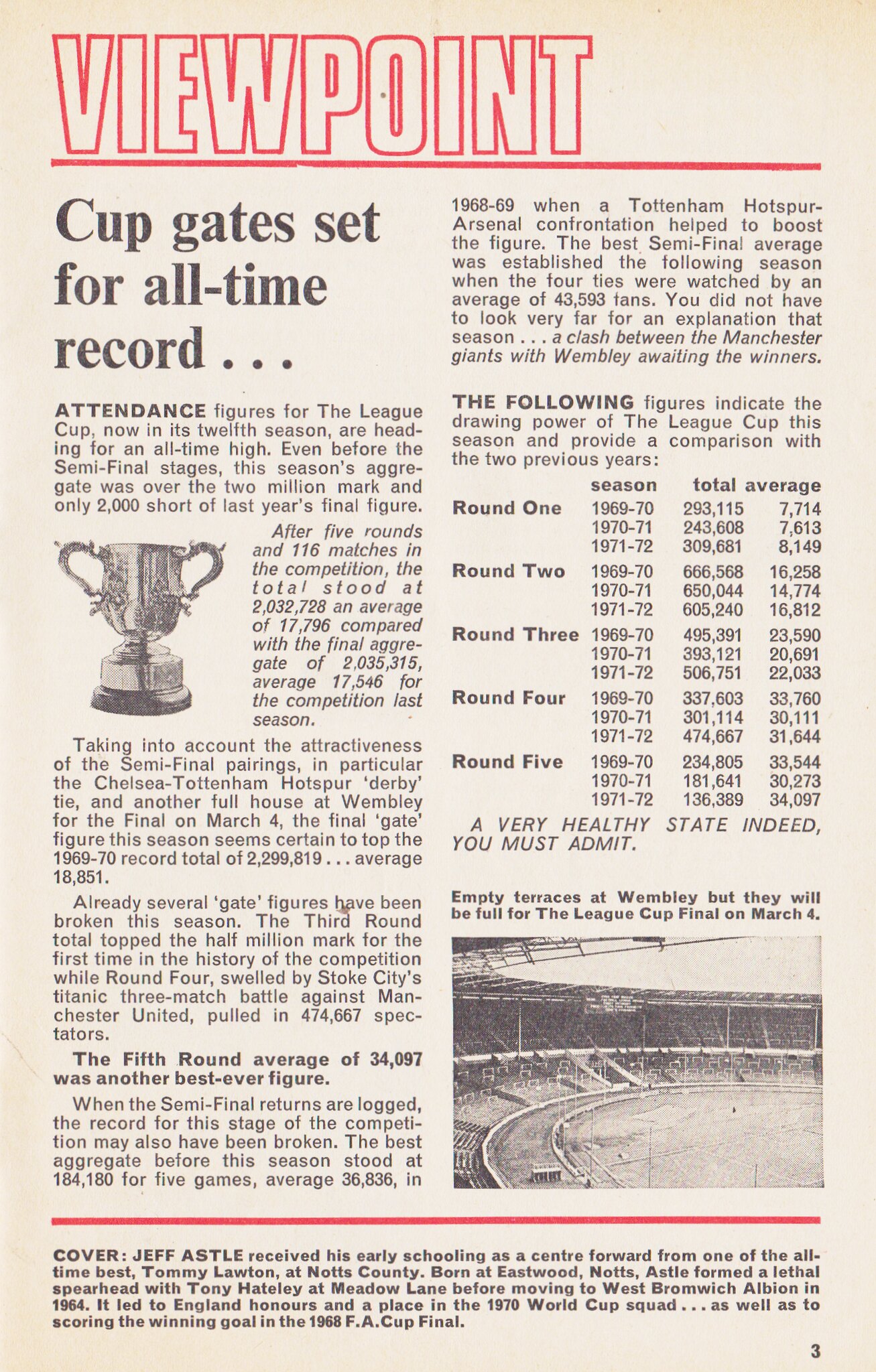The image is a scan of a vintage newspaper or magazine article that appears aged with a light tan or pinkish background. The article is titled "Cup Gates Set for All-Time Record" and focuses on the record-breaking attendance figures for the League Cup in its 12th season. At the very top of the page, the word "Viewpoint" is prominently displayed in bold white font outlined in red, followed by a solid red line running horizontally across the width of the page.

The article is divided into two columns of text, detailing how the League Cup's attendance has surged past the two million mark even before the semifinal stages, narrowly missing last year's final figure by only 2,000 spectators. Across the five rounds and 160 matches, the competition has drawn a total of 2,032,728 attendees, with an average of 17,796 per match, compared to the previous year's total of 2,035,315. Various records for attendance were broken, notably in the third and fourth rounds, with significant matches such as Stoke City's rematch against Manchester United drawing large crowds.

In the middle left of the article, there is an image of a football trophy breaking up the text columns. At the bottom right corner of the page, there is a faint page number, '3'. On the bottom left, there's an image of an empty stadium with faded terraces, accompanied by a caption indicating that it will be full for the League Cup final on March 4. 

Below this is additional text containing historical context, referencing individual players and their contributions, including Jeff's early schooling as a center forward under Tommy Lawton at Notts County and his subsequent career achievements. The article is framed by red borders at the top and bottom, giving it a structured and formal appearance.